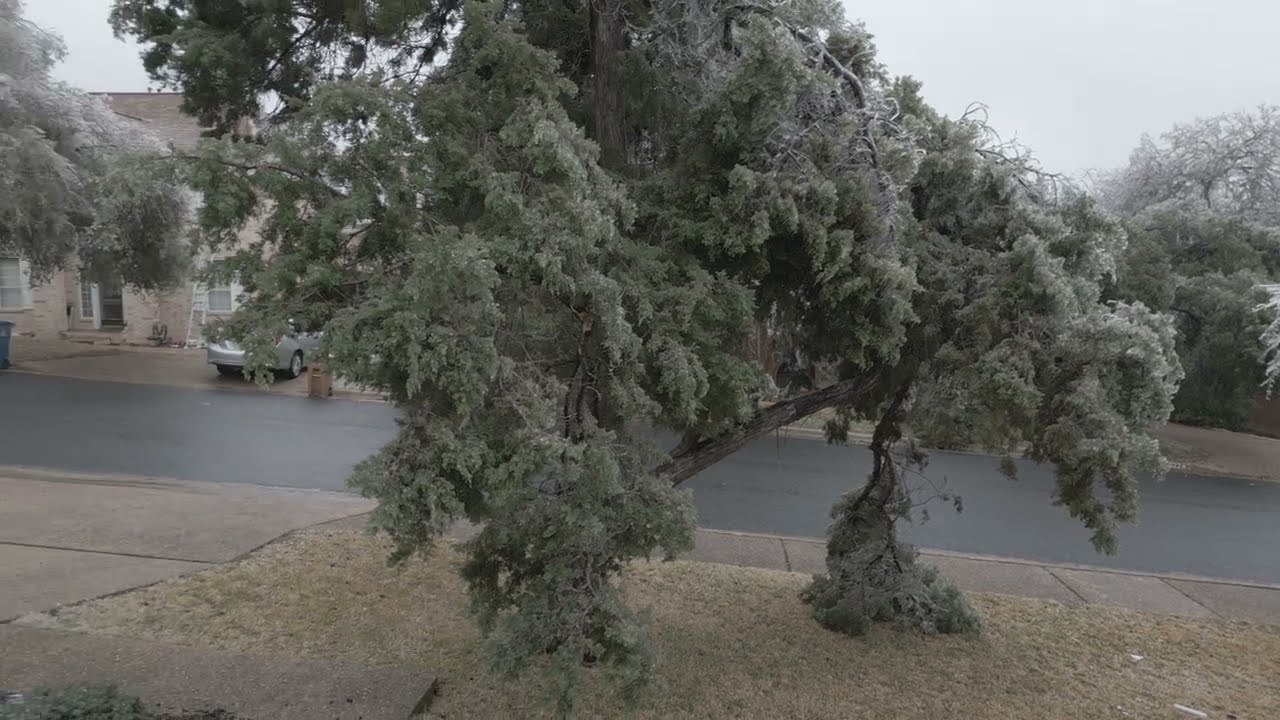This outdoor photograph, taken on a cloudy or rainy day, captures a scene from a residential neighborhood in horizontal landscape orientation. The focal point is two large trees with heavily canopied, green leaves that appear wet and drooping, likely from recent rain. These trees grow from a grassy front lawn in the foreground, bordered on the left by a paved cement driveway. Just beyond the trees, a wet, shiny asphalt road and a cement sidewalk are visible.

Across the road, partially obscured by the trees in the foreground, stands another residential building with a driveway. A silver car is parked in the driveway, and a blue garbage can and a piece of furniture are placed by the curb. The upper left center of the image provides a glimpse of a rooftop with white-trimmed windows and a door, suggesting a stone building. A white ladder leans against the building, and the tan-colored roof can also be seen through the foliage.

In the upper right corner, a distant tree line shrouded in misty clouds is visible, with a gray and overcast sky above, adding to the overcast ambiance of the photograph. The scene is bathed in daylight, ensuring clear visibility despite the gloomy weather.